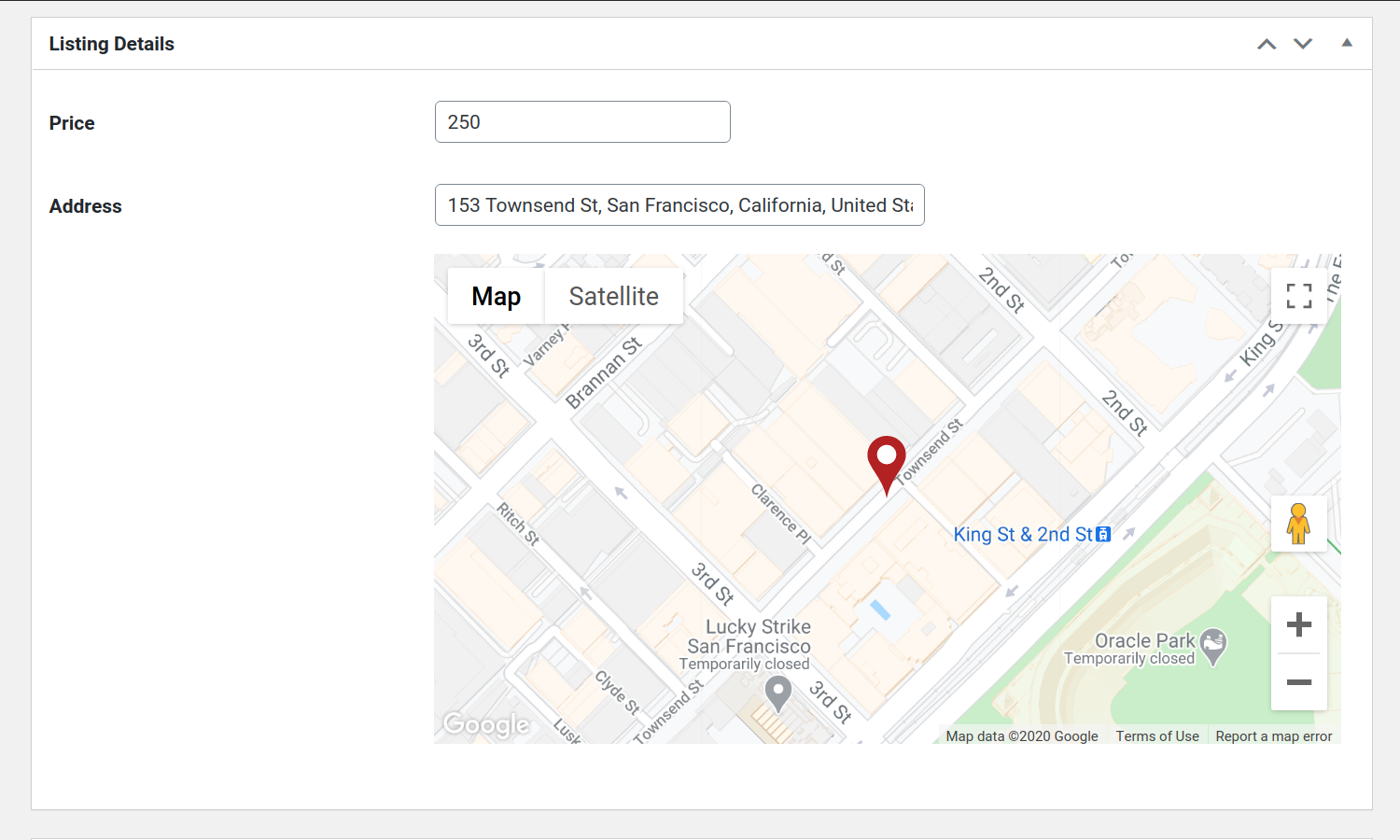The image is a screen capture of a real estate listing interface featuring a map. In the upper left-hand corner, the title "Listing Details" is prominently displayed. To the far right, there are an up arrow, a down arrow, and a small gray triangle. Below "Listing Details" runs a horizontal line that extends beneath these icons.

Directly under this line, the word "Price" is shown, accompanied by an input box containing the number "250." Below "Price" is the word "Address," which is in black font and also features an adjacent input box. The address in this box is "153 Townsend Street, San Francisco, California, United States."

Taking up the majority of the image is a detailed map, pinpointing the location of 153 Townsend Street with a distinct red icon featuring a white circle at its center. Options to switch between "Map" and "Satellite" views are available, along with plus and minus buttons for zooming in and out. In the bottom right-hand corner of the map, icons indicate the availability of terms of use and report functionality for map errors.

The background of the image is entirely white, with no other text or images that draw attention.